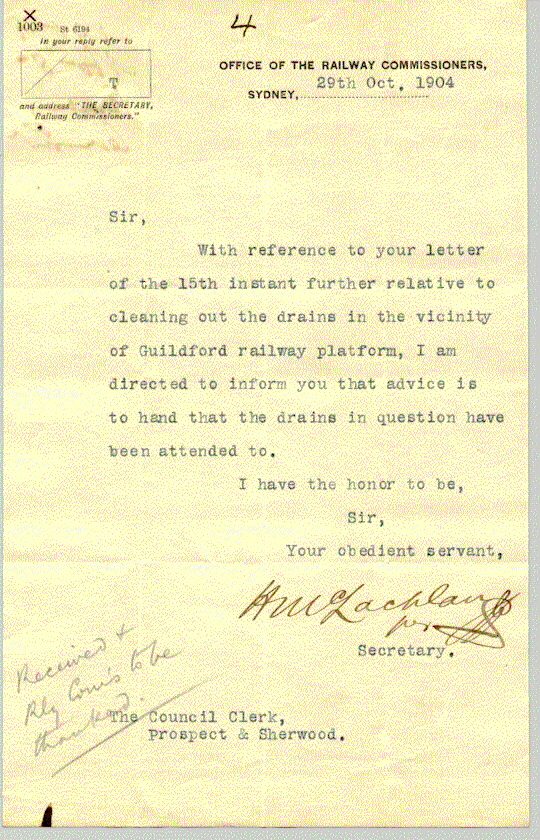This image depicts a photograph of a historic document, specifically a letter from the Office of the Railway Commissioners, Sydney, dated 29th October 1904. The paper has aged to a faded, almost pinkish-yellow hue with a slightly rough texture, and a white background is faintly visible behind it. At the very top, a handwritten number '4' appears alongside a designated space in the upper left corner, likely intended for stamps or additional notes. The heading on the upper right reads, "Office of the Railway Commissioners, Sydney," followed by the date stamp "29th October 1904."

The letter is typewritten and begins formally with "Sir," referencing a previous letter dated the 15th of the same month. It discusses matters related to the cleaning of drains near the Guildford Railway Platform, stating, "I am directed to inform you that advice is to hand that the drains in question have been attended to." The closure reads, "I have the honour to be, Sir, your obedient servant," followed by an illegible cursive signature with the title "Secretary" beneath it. At the very bottom, a typed notation reads, "The Council Clerk, Prospect and Sherwood," with a handwritten note indicating that the letter was reviewed.